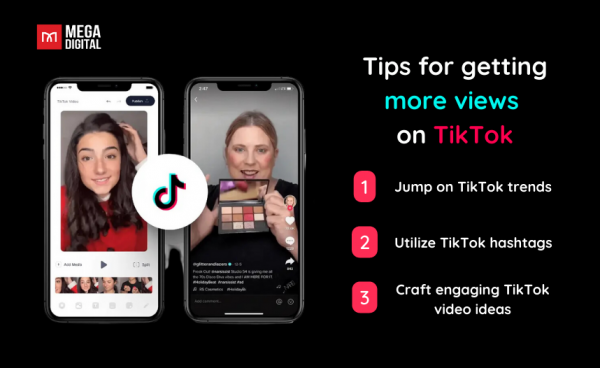**Advertisement for Megadigital: Tips for Boosting Your TikTok Views**

On a solid black background, the advertisement prominently features the branding of Megadigital. In the top left corner, a striking red square with a white letter 'M' sits beside the site name, "Megadigital," in bold white letters.

The left side of the image showcases two black cell phones placed side by side, each screen displaying a TikTok video. Between the phones, a round circle bears the TikTok logo.

To the right of the phones, the ad lays out three essential tips for increasing TikTok views:
1. **Jump on TikTok trends** (highlighted in a red square).
2. **Utilize TikTok hashtags**.
3. **Craft engaging TikTok video ideas**.

The screen of the left phone features a woman with long black hair wearing a red shirt, while the right phone displays a woman with her hair pulled back, holding a colorful makeup palette in both hands, presented close to her face.